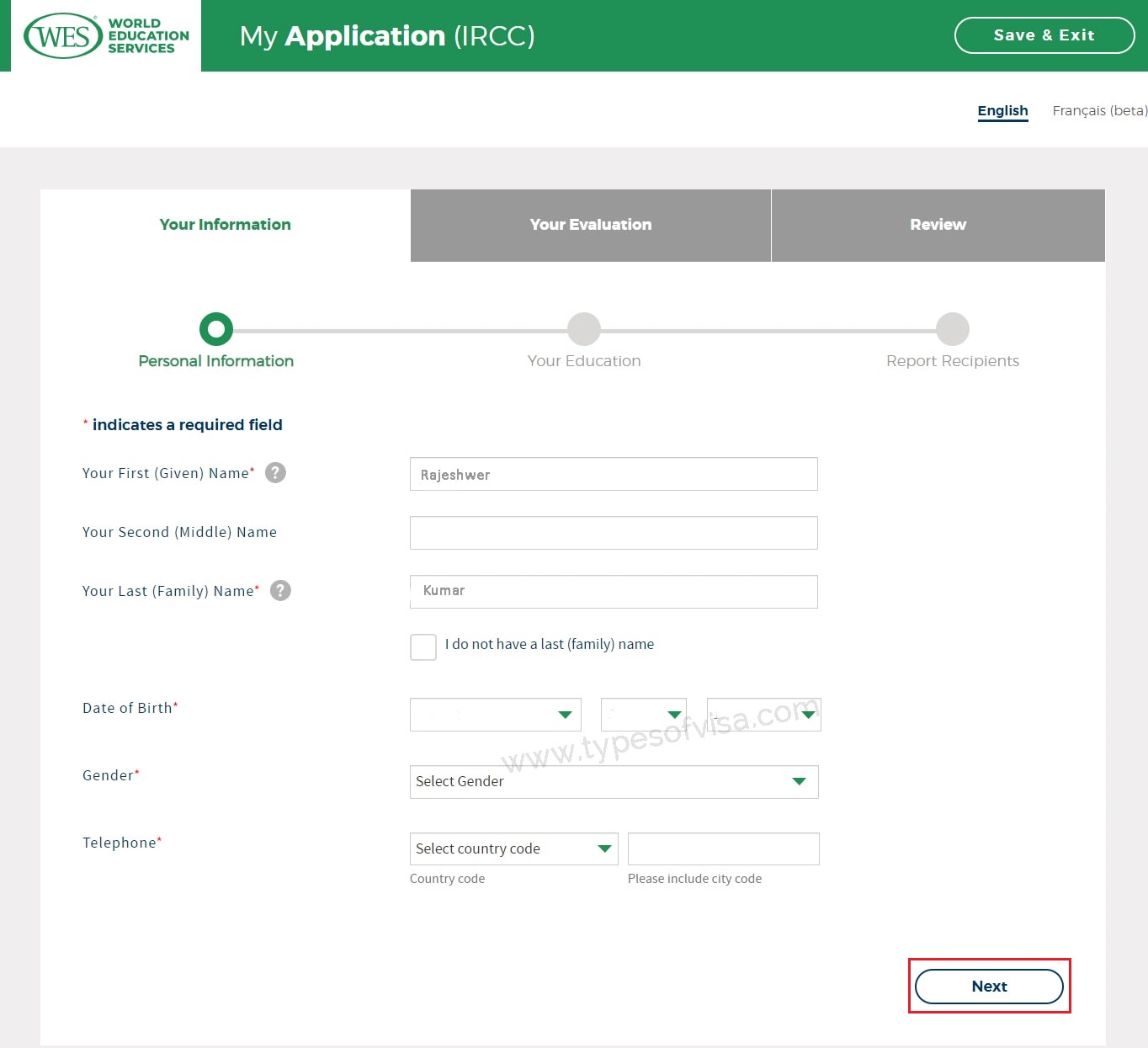This image captures a detailed view of the World Education Services (WES) website. At the top left corner, there is an oval logo with a green border containing the capital letters "WES." To the right of the logo, "World Education Services" is written in a small, bold, green, capitalized font. Directly below, a green strip features a headline that says "My Application" where "My" is in white non-bold font and "Application" is in bold white font. To the right of the headline, the acronym "IRCC" is enclosed in parentheses, written in an unbolded font.

Further to the right, a white-bordered oval with a transparent background blends into the green and white strip, featuring the words "Save and Exit." Below this, there is a white strip with an option to select the website language; "English" is underlined in dark blue, indicating it is clickable, followed by the French option.

The main section of the screen has a light gray background with three clickable options arranged horizontally. The first option, "Your Information," is highlighted in white with green text, signifying it is selected. To the right, additional options "Your Evaluation" and "Review" are displayed with a medium gray border and bold, white text, contrasting the selected green-highlighted option.

In the bottom right corner, there is an oval-shaped "Next" button outlined in black with black text. It is prominently bordered by a red rectangular outline, indicating it is the active button to proceed to the next step.